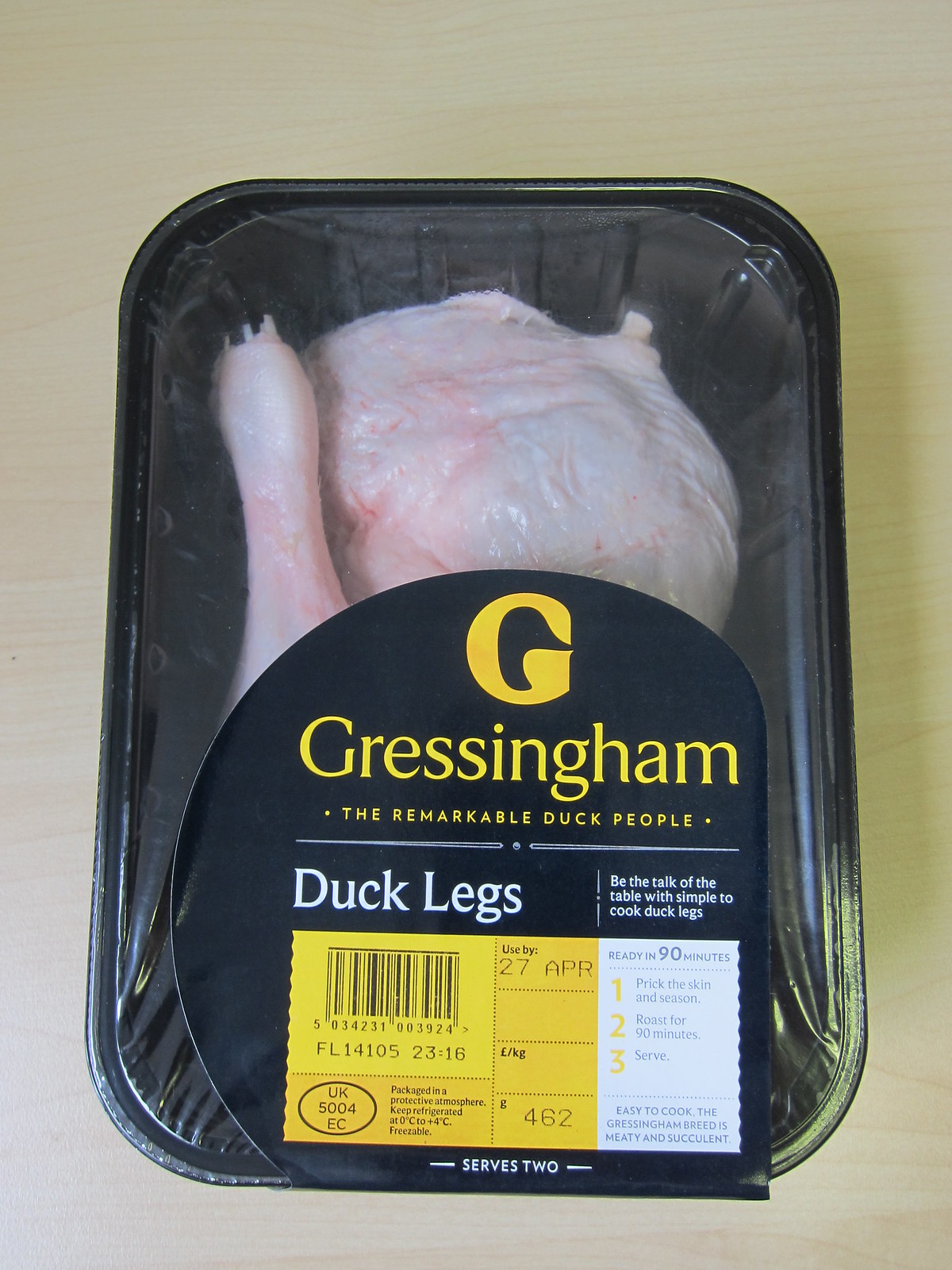This is a detailed photograph of a supermarket-packaged meat product, specifically duck legs by Gressingham, "The Remarkable Duck People." The product lies on a wooden counter, encased in a clear vacuum-sealed plastic wrapping that reveals the pink and white hues of the meat inside a black tray. Dominating the package is a large black sticker featuring the brand's logo: a prominent yellow 'G' and the company name "Gressingham" in white text. The label provides extensive information, including cooking instructions that recommend pricking the skin, seasoning, roasting for 90 minutes, and serving, making it simple to cook these succulent and meaty Gressingham duck legs. The price is listed as $4.62, though the currency type is unclear. Additional details include a use-by date of April 27th, no year specified, weight and product specifics, a yellow UPC code, and the code UK 5004 EC.